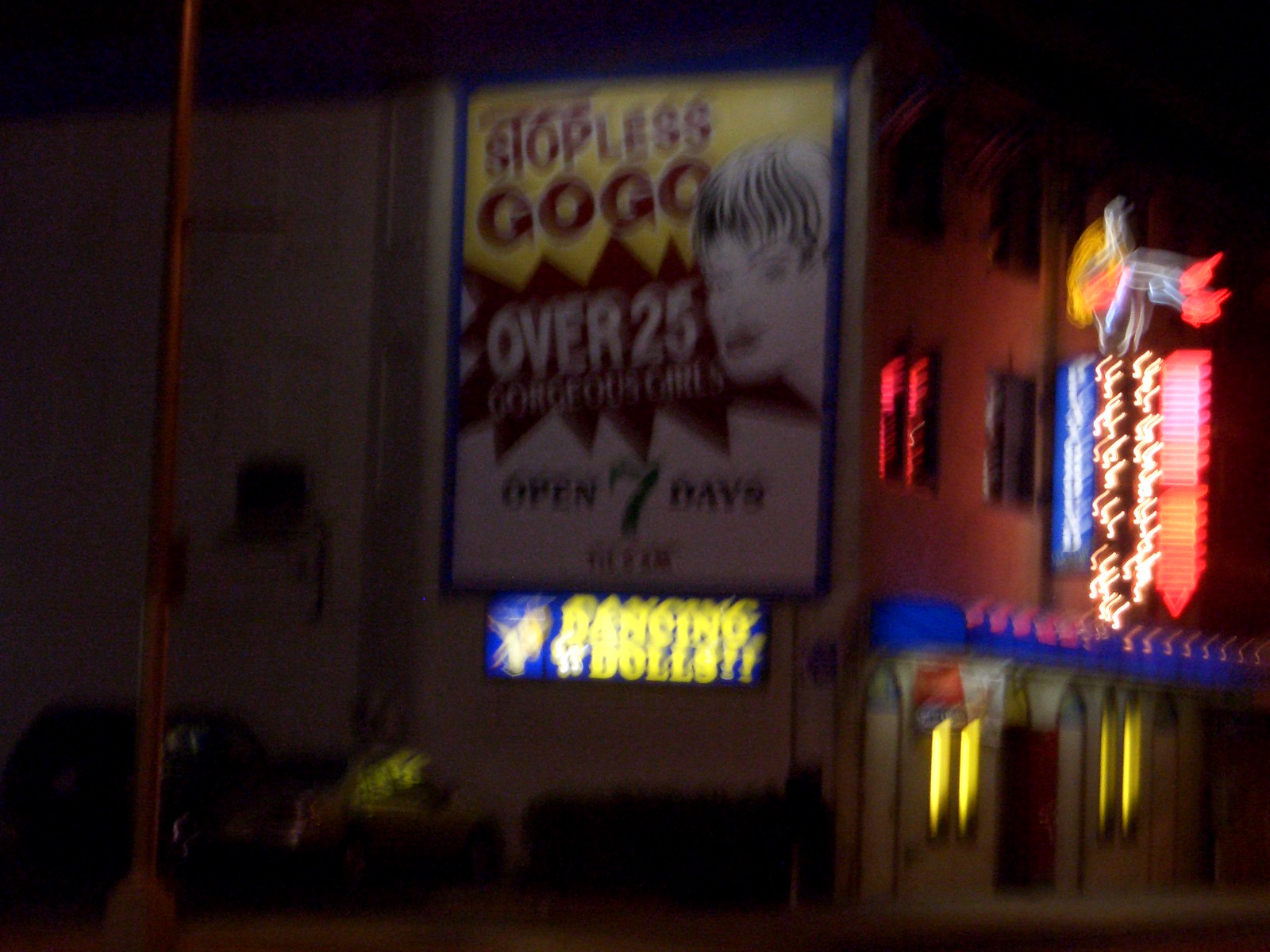In this extremely blurry nighttime photograph, the main focus is a three-story commercial building, possibly a gentleman's nightclub or adult club, situated in a city. The sky in the background is pitch black, contributing to the overall darkness of the scene. Dominating the image is the side and front view of the building, adorned with numerous neon lights and signs.

On the side of the building, a large, illuminated billboard features a woman with fair skin, red lipstick, and short black hair. The billboard text, though partially obscured, reads: "Stopless Go-Go, over 25 gorgeous girls, open seven days a week." Beneath this billboard is a smaller, blurry sign that reads "Dancing Dolls." Additional neon signage and arrows point downward, guiding attention toward a blue awning at the building's entrance, which is flanked by yellow lights.

The building has several windows, most of which are dark except for one on an upper floor bathed in red light from within. On the left side of the photograph, a dark-colored van can be discerned, though details are obscured due to both shadow and the overall blurriness of the image. Despite the poor quality of the photo, the bright neon lights and signage hint at the building's possible use as an adult entertainment venue.